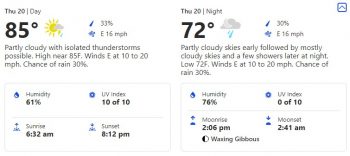**Detailed Weather Forecast for Thursday, 20th**

**Daytime Forecast:**
- **Date:** Thursday, 20th
- **Temperature:** High of 85°F
- **Weather:** Partly cloudy with isolated thunderstorms possible
- **Precipitation:** 30% chance of rain with a possible 33% index (not entirely sure what this indicates)
- **Winds:** East at 10 to 20 mph
- **Humidity:** 61%
- **UV Index:** 10 out of 10
- **Sunrise:** 6:32 a.m.
- **Sunset:** 8:12 p.m.

**Nighttime Forecast:**
- **Date:** Thursday, 20th
- **Temperature:** Low of 72°F
- **Weather:** Partly cloudy skies early followed by mostly cloudy conditions with a few showers later at night
- **Precipitation:** 30% chance of rain
- **Winds:** East at 10 to 20 mph
- **Humidity:** 76%
- **UV Index:** 0 out of 10
- **Moonrise:** 2:06 p.m.
- **Moonset:** 2:41 a.m.
- **Lunar Phase:** Waxing Gibbous Moon